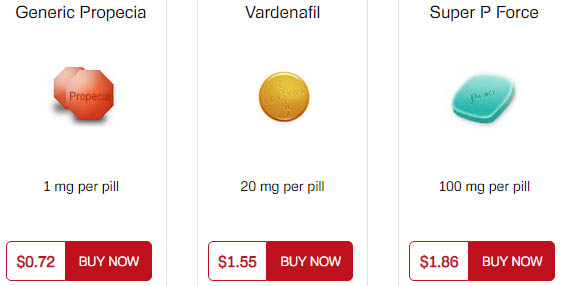This screenshot captures a segment of a webpage dedicated to selling various types of pills, each presented in its own clearly defined column. 

In the leftmost column, the product featured is "Generic Propecia." Beneath its name, two animations depict the pill as red octagons, each emblazoned with the word "Propecia." The dosage information reveals that each pill contains 1 milligram of the active ingredient. A "Buy Now" button is conveniently placed below, displaying the price of $0.72 per pill.

The middle column showcases "Vardenafil." The visual representation shows a yellow, circular pill. This medication is available in 20 milligrams per pill. Similar to the previous column, a "Buy Now" button is positioned underneath, indicating a price of $1.55 per pill.

In the rightmost column, "Super P Force" is highlighted. The pill is depicted as a blue, diamond-shaped tablet. The dosage for this medication is specified as 100 milligrams per pill, accompanied by a "Buy Now" button listing the price of $1.86 per pill.

Each column provides a clear and concise overview of the pill, including imagery, dosage, and pricing, making it easy for potential buyers to compare and make informed decisions.